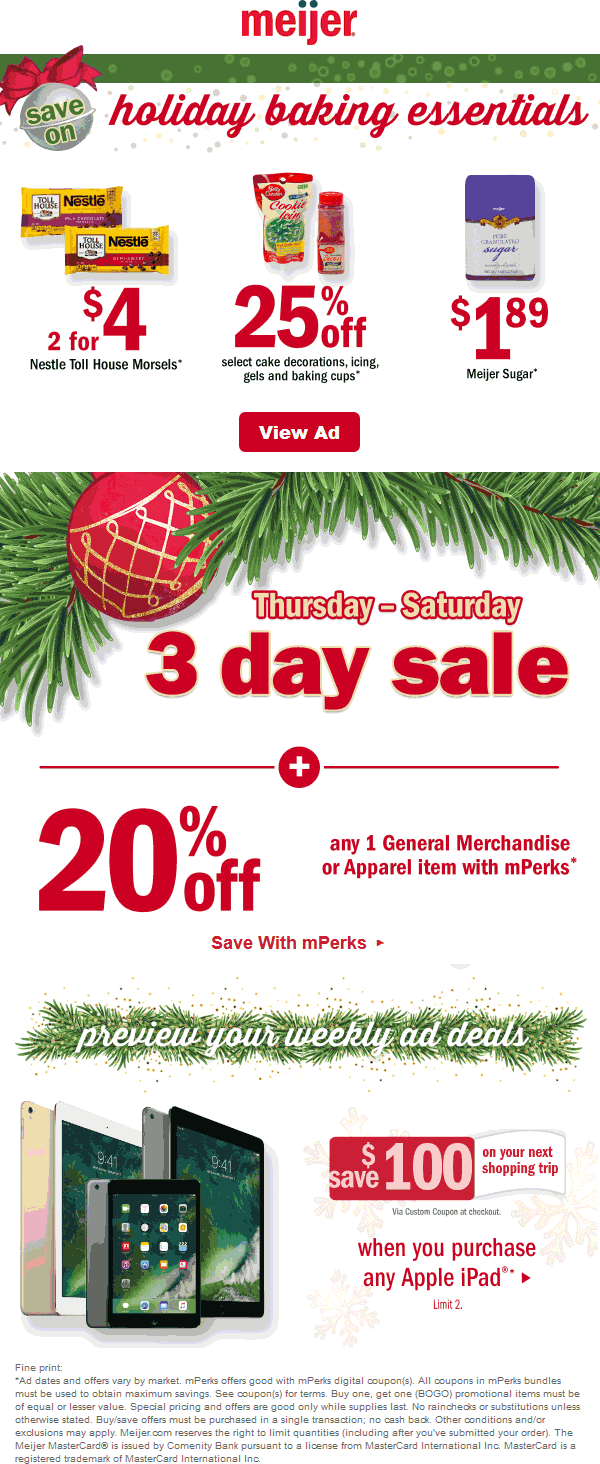**Detailed Caption:**

The image is a vibrant holiday advertisement that prominently features the brand "Major" written in red text with two green dots accentuating the 'i' and the 'j'. The ad is promoting "Holiday Baking Essentials" with a headline text, followed by "Save on $2.44 Nestle Chocolate Chip Cookies or Morsels". Adjacent to this, "25% off select cake decorations" is highlighted in red text, alongside "Major Sugar" displayed in white and blue packaging for $1.89.

In the center, a red button with the text "View Ad" stands out against a background of green foliage adorned with a red Christmas ornament, reminiscent of a Christmas tree. Below, the ad details a "Thursday - Saturday Three-Day Sale" separated by a red line with a white plus symbol in a circle at its midpoint.

At the bottom, "20% off any one general merchandise or apparel item with mPerks" is mentioned, including a note to save with mPerks. Further down, a green Christmas graphic with white text invites viewers to "Preview your weekly ad deals."

To the right, images of three iPads — two 10.9-inch models and one smaller iPad Mini — are featured. The ad promises "Save $100 on your next shopping trip when you purchase any Apple iPad" with small gray text below offering additional deal details.